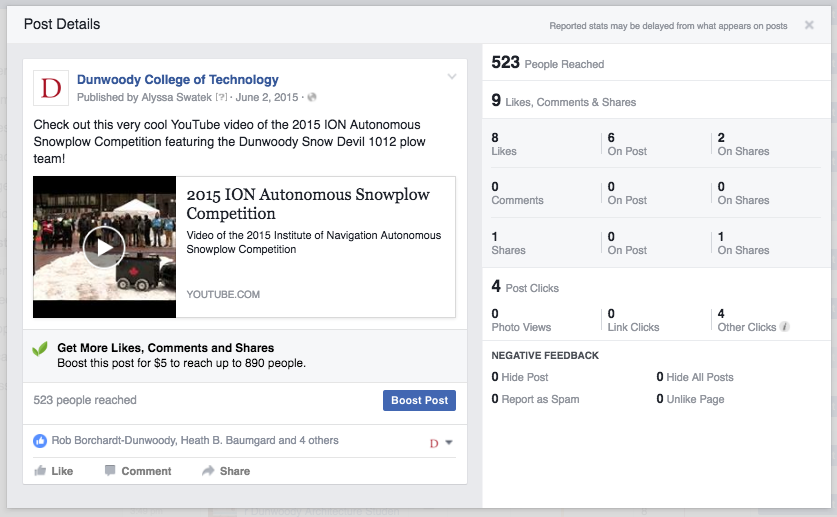This image is a comprehensive screenshot showcasing the statistics and engagement tracking for a Facebook post published by Dunwoody College of Technology. 

At the top left corner of the screenshot, the "Post Details" section is prominently displayed in bold, followed by reported statistics on any delayed appeals associated with the post on the far right. The detailed information below includes the post's publication date, June 2, 2015, and the publisher, Alicia Schnavek.

The main content of the post highlights a YouTube video featuring the 2015 Iowa and Autonomous Snow Plow Competition team, specifically mentioning Dunwoody's "Snow Devil, 10-12 Plow Team." The post promotes the video, encouraging viewers to "check out the story."

Further down the screenshot, there's an option to boost the post for $5 to enhance its reach up to 880 people, with a "Boost Post" button located on the right. As of the screenshot, the post has reached 523 people.

The engagement metrics are broken down as follows:
- **Reach:** 523 people
- **Interactions:** 
  - **Likes, comments, and shares:** 9 total
  - **Likes:** 8 (6 on the post, 2 on shares)
  - **Comments:** 0
  - **Shares:** 1 (1 on the post)
- **Post Clicks:** 4 (comprising 4 photo views and 0 other clicks)

Additionally, negative feedback metrics indicate zero instances of the post being hidden, marked as spam, or the page being unliked.

Overall, this image is a vivid example of a statistical tracking program used to monitor and analyze Facebook post engagements and reach for Dunwoody College of Technology's publications.